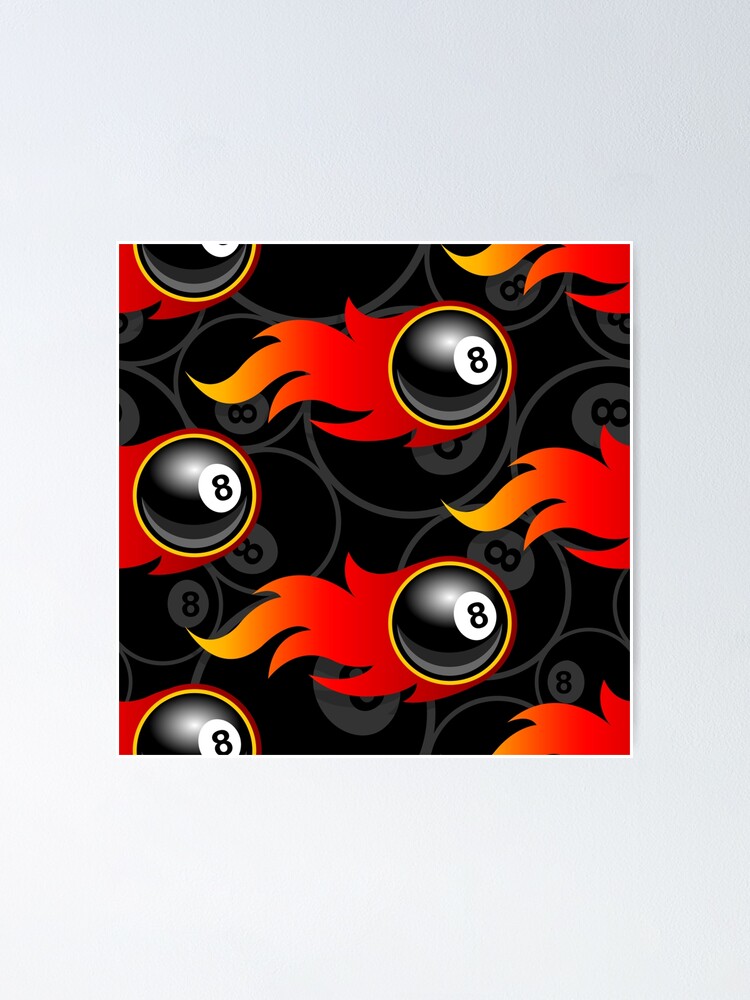The image is a graphic, likely intended as a wallpaper for devices like cell phones or desktop computers. It features a repeating design of stylized 8-balls typically found in billiards, with a vivid fiery motif trailing behind each ball. The primary 8-balls are sharp and detailed, each encased in a traditional white circle with the number eight. They are surrounded by flames that transition from bright red near the ball to orange and finally yellow at the tips, giving the impression of movement from left to right. 

In contrast, the background is black, adorned with faded, grayed-out 8-balls of various sizes, enhancing the sense of depth and filling the negative space without competing with the foreground elements. The fiery tails resemble stylized Asian dragon or koi fish designs, adding a dynamic, almost mythical quality.

The design is continuous, ensuring that when set as a wallpaper, it extends seamlessly across the screen. This visually striking and cartoony style, with its bold colors and directional flow, is likely meant to capture attention and add a vibrant, animated feel to whatever surface it adorns.